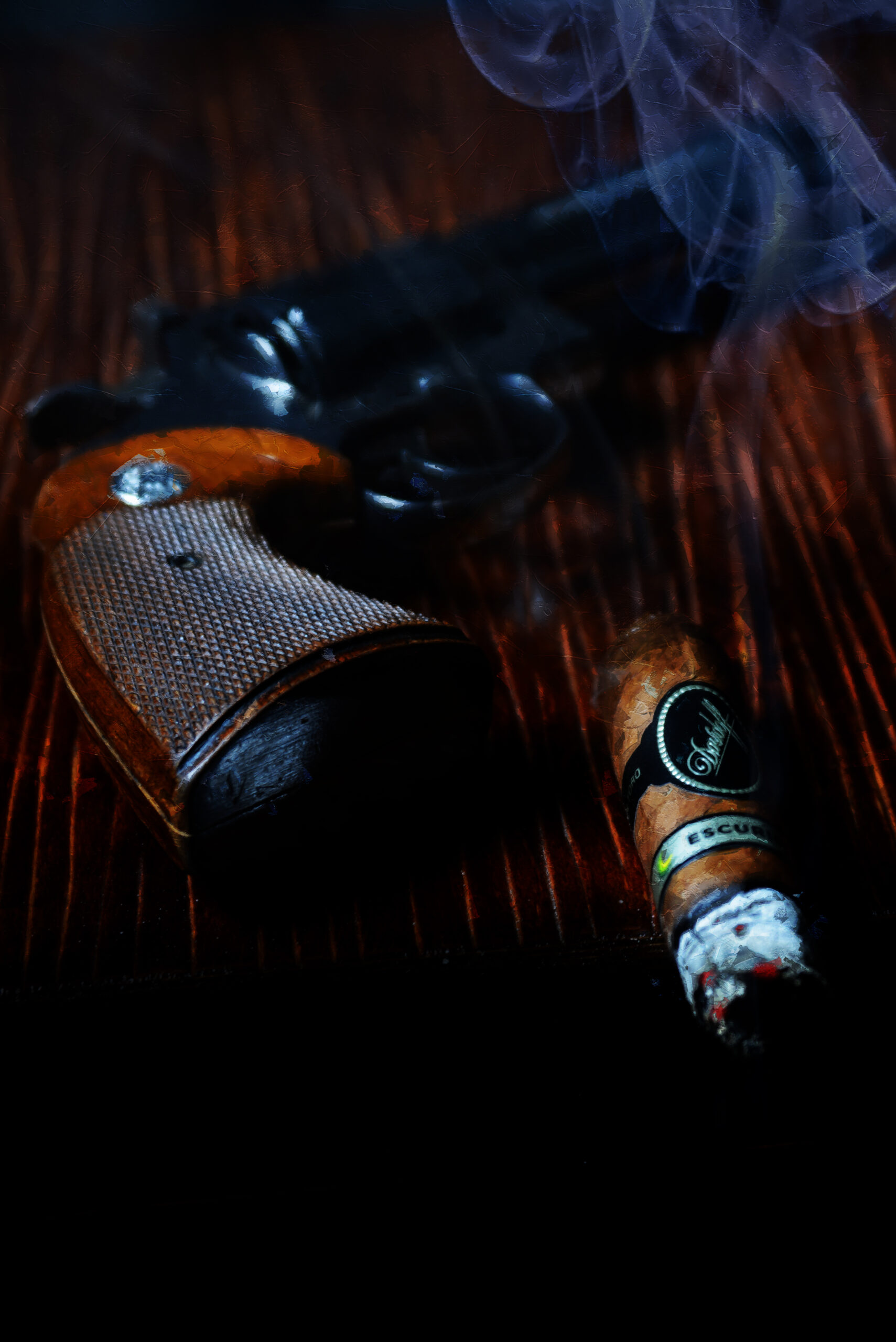The image depicts a close-up, artistic composition of a short-barreled revolver with a brown, wooden grip, and a lit cigar. The gun, featuring detailed elements like a screw and possible jewel above the handle, is positioned against a dark, moonlit-like background that contrasts with the dark wooden surface it's laid on, possibly a nightstand. The cigar is partially burnt, revealing orange ashes and a smoldering tip, accompanied by swirling smoke that drifts towards the upper right corner, exhibiting a subtle blue or periwinkle hue. The cigar also has an unreadable brand label. The overall scene exudes a mysterious, stylistic ambiance, focusing intently on the interplay between the gun and the cigar.